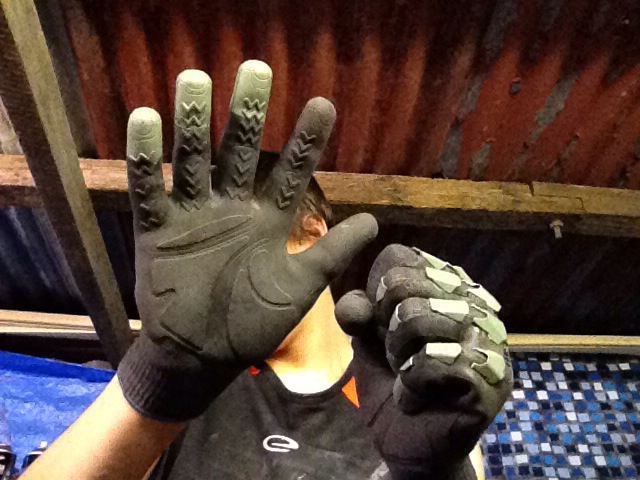The photograph captures a person with their face obscured by gloved hands, preventing clear identification of their gender. The gloves, black with a combination of white padding and reinforced sections, feature distinct details: the left hand clenched into a fist and the right hand held open with fingers widespread. The right glove has white padding on the middle, ring, and pinky fingers, while the thumb and index finger remain unpadded. The person wears a black t-shirt with orange epaulette-style designs on the shoulders and a white letter 'E' in the center. The photo is taken from a slightly low angle, allowing a view of the rusted red corrugated metal roof supported by wide brown wooden beams. The background also includes blue walls and a mosaic of dark blue, light blue, and white tiles. The image suggests that the person might be a worker who does not want their face shown. The overall composition, with the protective gloves and the mixed textures and colors of the surroundings, conveys a gritty and industrious atmosphere.